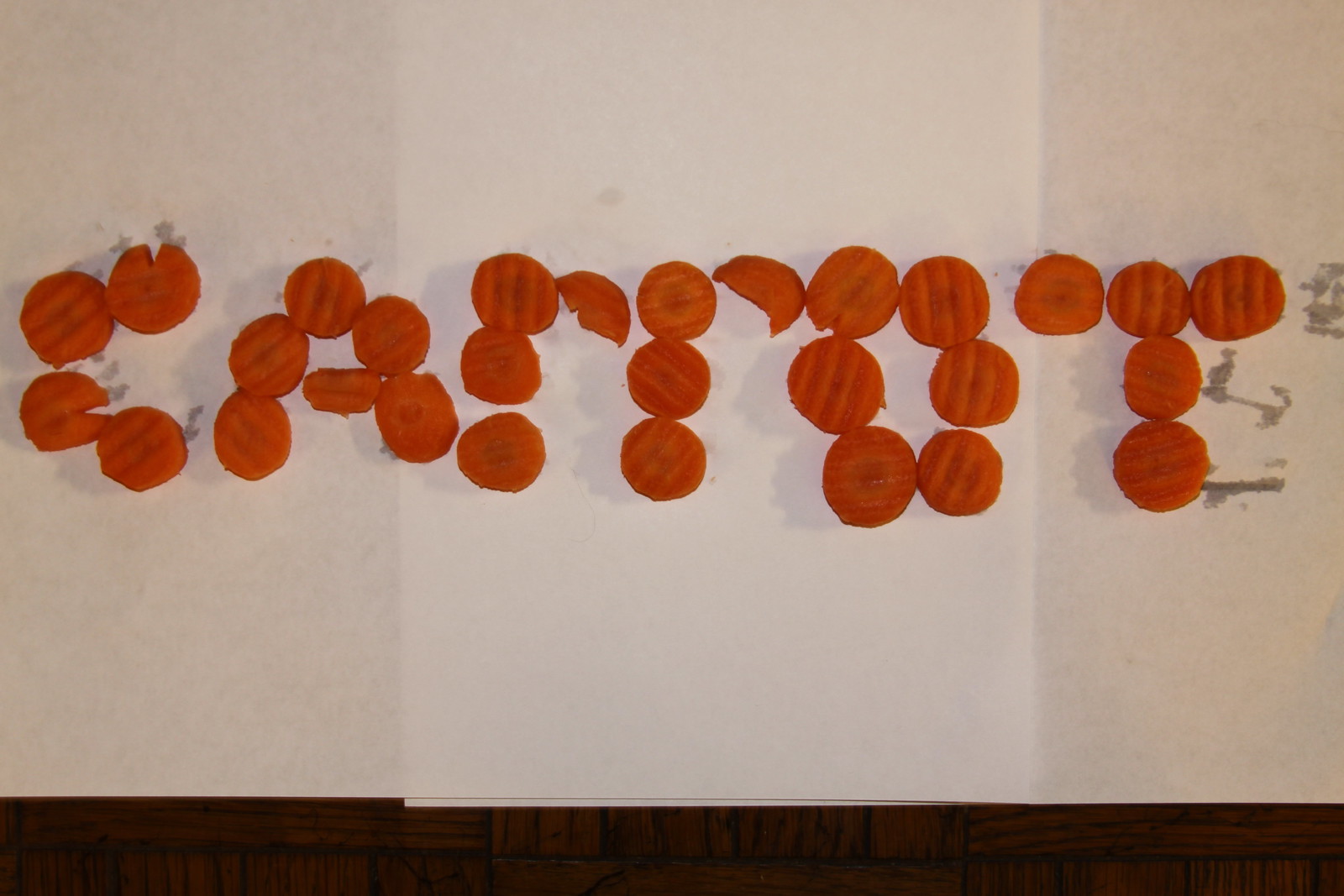This indoor color photograph is a top-down, close-up image of a collection of carrot slices intricately arranged on white notebook paper to spell out the word "carrot" from left to right. The carrot slices, approximately an inch and a half in diameter, are uniformly cut and feature ridges, suggesting they were sliced using a specialized slicer rather than a regular knife. The meticulous arrangement includes thoughtful use of semi-circular slices to form the curved part of the letter "R". In total, around 20 to 25 carrot slices are used to create the letters: four slices for "C", six for "A", three and a half each for the two "R"s, six for "O", and five for "T". The white notebook paper has some water stains on the right side, and the background transitions to a dark, possibly parquet floor or another wooden surface. Despite the focused nature of the image, it is poorly lit, appearing slightly dark, with no other text or wording present.